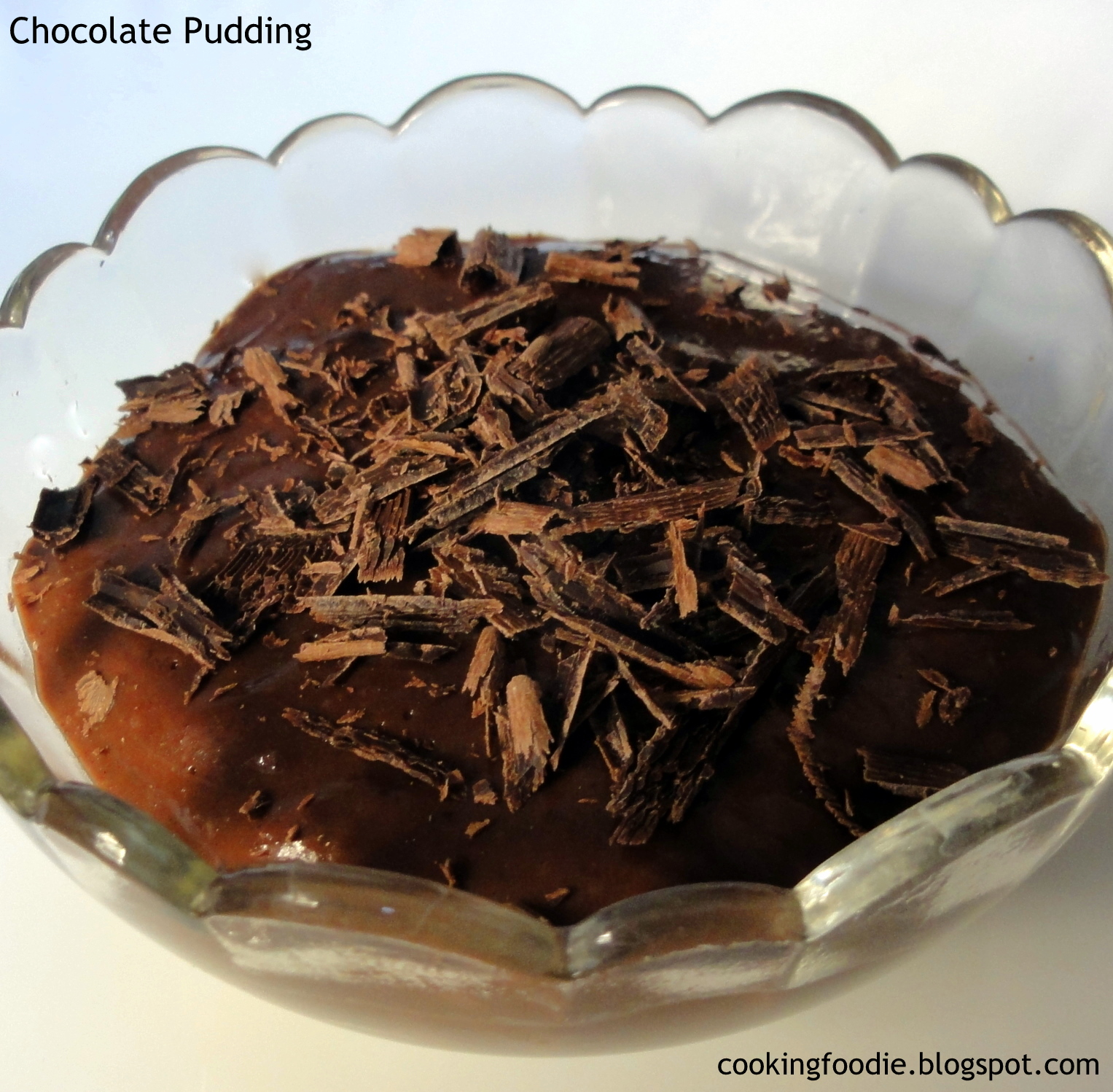In this close-up photo, an elegant glass bowl, styled with petal-like curved edges reminiscent of a 1950s design, takes center stage on a countertop, devoid of any background distractions. The glass bowl cradles an opulent and creamy chocolate pudding, generously topped with rich chocolate shavings that enhance its luxurious appeal. In the upper left corner of the image, the words "chocolate pudding" are inscribed in black text, while the bottom right corner features the source "cookingfoodie.blogspot.com." The textured chocolate topping and ornate bowl collectively emphasize the dessert's indulgent and homemade quality, inviting viewers to savor its visual allure.